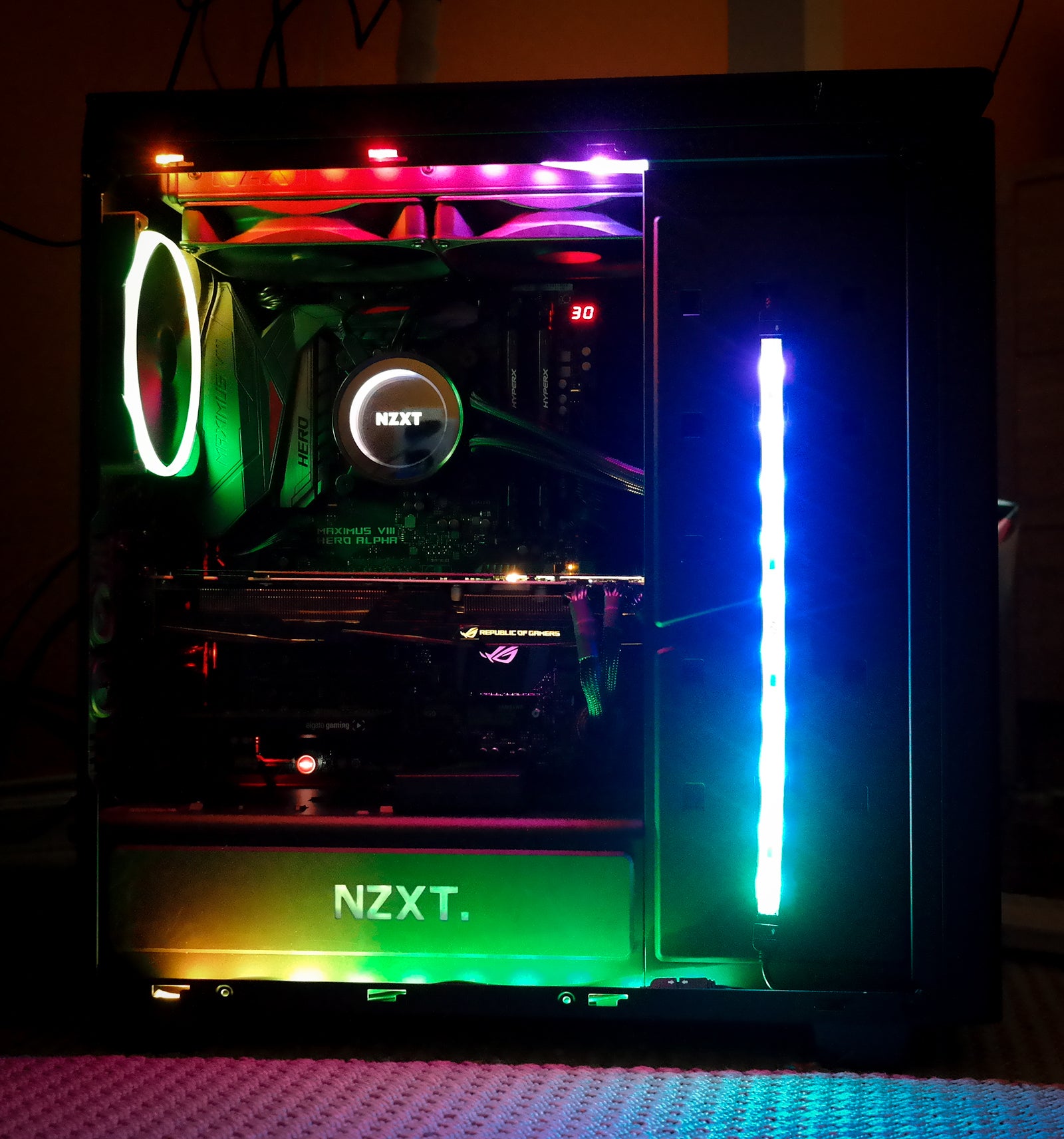This photograph, taken in the dim ambiance of a dark room, showcases a large, futuristic NZXT gaming tower radiating vibrant neon lights. The prominent NZXT logo is displayed twice, once along the bottom panel and again higher up on a circular component. An eye-catching vertical LED strip of cool white and bluish tones illuminates the right side of the tower, contrasting with an array of additional lights in hues of orange, red, purple, and green spread across the structure. Inside, the tower's intricate wiring and components are visible, highlighted by a bright white ring light and accented with pink and purple neon. A red digitized number "30" stands out on the upper right portion. The device, made of sleek metal, rests on a textured gray floor, and the background wall exudes a muted orange-gray color, both elements adding to the high-tech atmosphere of the scene.